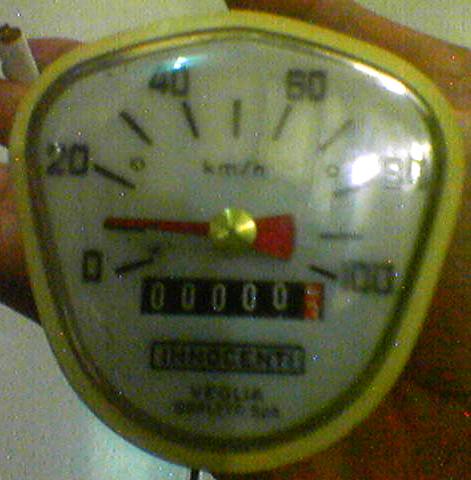The image depicts a vintage speedometer, likely from several decades ago, and appears blurry due to poor photo quality and low lighting. The small, circular speedometer features what seems to be a brass metal outline, though it could merely be reflecting light, giving it a brassy appearance. The gauge face is marked with numbers ranging from 0 to 100, with increments marked at 20, 40, 60, and 80 km/h, indicating that the unit measures speed in kilometers per hour. A red needle, anchored by a brass or gold centerpiece, points to the speed reading. Below the needle, there is a manual mileage tracker currently displaying zero miles. The speedometer face also includes a black rectangular label with the brand name "Innocenti" printed on it. Additional, indistinct text appears below the brand label, but it is too fuzzy to decipher clearly. A noticeable, blurry white reflection, potentially from a window, obscures part of the image. In the foreground, a hand holding a cigarette grips the speedometer, adding a human element to the composition.